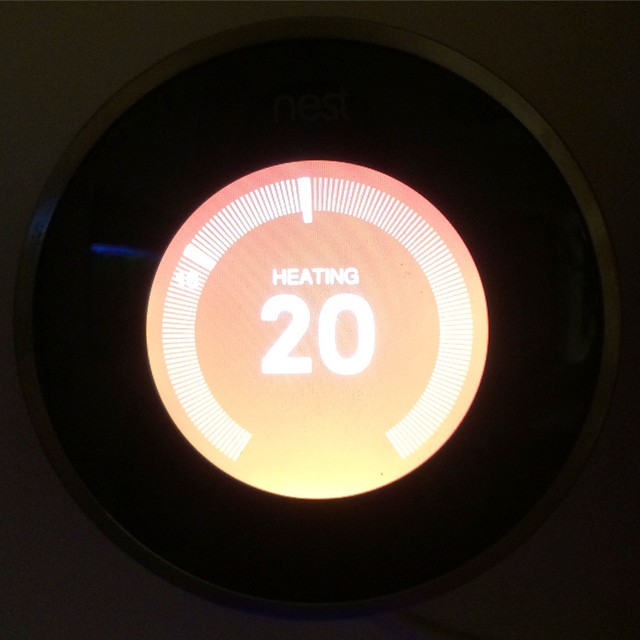This photograph captures a close-up view of a sophisticated data display instrument, possibly from a vehicle dashboard or a heating system interface, set against a black background. Central to the image is a prominent peach-colored circular display encircled by a thick black ring and a thin brown or black line. The circle exhibits a gradient, transitioning from peach at the top to yellow at the bottom, with yellow stripes piercing through the middle. Surrounding the main circle are numerous thin lines encompassing the display, with two notably thicker lines among them. Below one of these thicker lines is the number "18."

Bright blue light emerges from the left side, casting an additional hue over the display. Prominently featured in the center of the display are the capitalized word "HEATING" and the number "20," suggesting this could be a control or indicator related to a heating function.